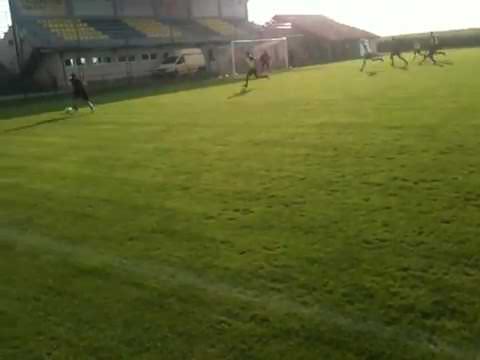The image depicts an outdoor soccer field, characterized by a continuous expanse of green without any visible line markings. In the midst of what seems to be a bright, sunny day, a group of around seven or eight players is seen congregating near the goal, which is situated towards the upper center of the image. The left-most player is in possession of the ball, appearing to have just reached it. 

The goalpost is set against a backdrop featuring a tiered seating arrangement with alternating blue (or possibly black) and yellow seats, elevated atop a structure that resembles a long garage or storage building. A white van, equipped with a camper shell, is parked in front of this structure, oriented towards the left. Additionally, the scene includes vague shapes and figures, emphasizing the blurry nature of the photograph. The sky is bright, further suggesting daylight, as the indistinct setting captures players actively engaged in a game of soccer.